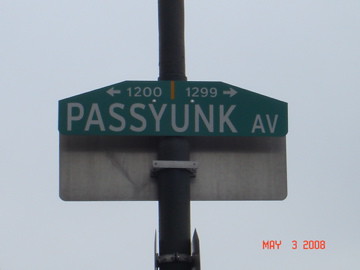This small, color photograph offers a close-up view of a road sign mounted on a tall black pole that runs vertically through the center of the image. The scene features two road signs installed back-to-back atop the pole. The foreground sign is dark green, with "1200" and a left-facing arrow on one side, and "1299" with a right-facing arrow on the other, both in smaller white font at the top. Below these numbers, large, bold white letters display "Passy Yonk AV." The backside of the second sign, barely visible above, is gray. The background of the photograph shows a gray, overcast sky, adding to the muted atmosphere. At the bottom of the pole, two small bars extend horizontally, the left one thinner than the right, connected by a horizontal bar. The photo is timestamped in the bottom right corner with the date "May 3, 2008" overlaid in red text.